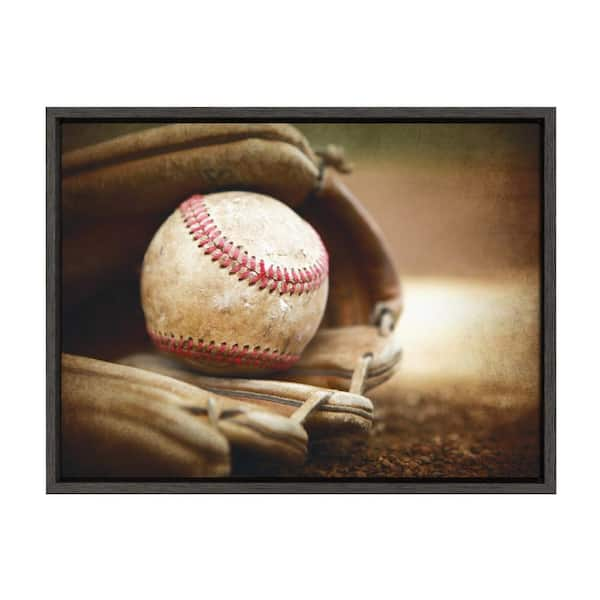This detailed close-up photograph captures a nostalgic, sepia-toned scene of a well-worn baseball cradled within an equally used brown leather catcher's mitt. The white baseball, adorned with red stitching, is stained extensively with mud and dirt, indicating it has seen many games. The baseball mitt, with cracked leather and lighter brown stitching, hints at its age and heavy use. One partially visible engraved letter, "S," on the mitt adds a layer of personal history to the image. The composition sits on a sepia-colored gravel ground, with blurred sepias, beiges, and greenish grays forming the background, enhancing the focus on the baseball and mitt. The dark gray border around the image gives it an older photographic feel, evoking a sense of time passed and the end of an era, perhaps metaphorically suggesting the game's end or the passage from one phase of life to another.